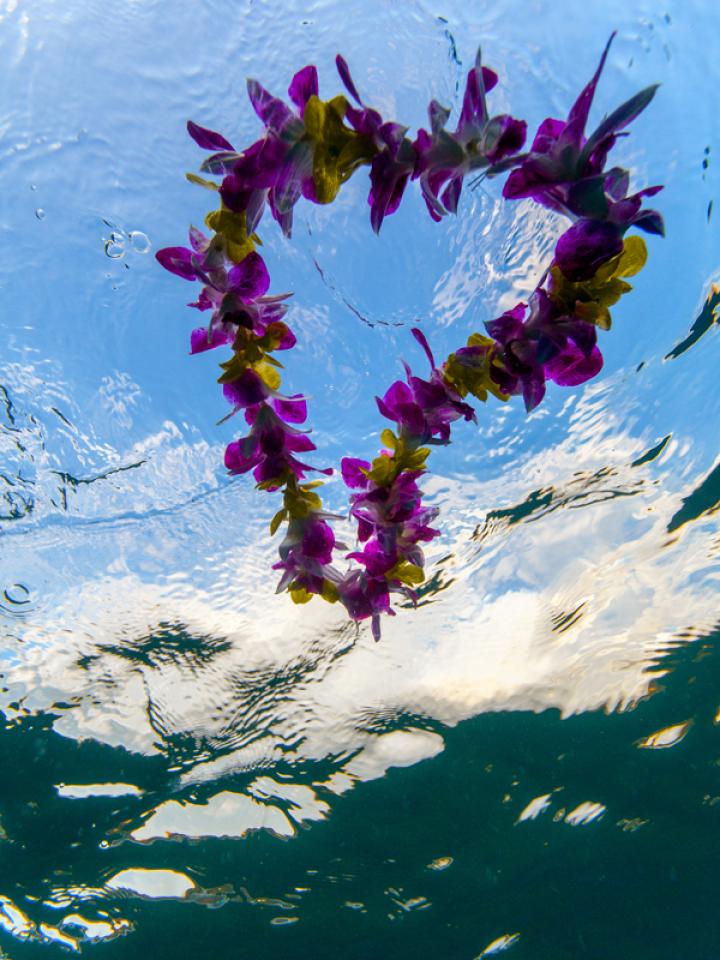An underwater photograph captures a vibrantly colored Hawaiian lei, predominantly composed of magenta, deep purple, and hot pink flowers interspersed with yellow flowers and green leaves, floating gracefully on the surface above. The lei, viewed from below, nearly forms a heart shape, adding a touch of whimsy to the scene. The water surrounding the lei exhibits a gradient of colors—from light blue at the top to dark green at the bottom, with a bright white center. Ripples and reflections dance across the water’s surface, revealing glimpses of the blue sky and scattered white clouds, while the sun’s indirect light casts the flowers in soft shadow, enhancing the mystery and depth of the image. The petals, some longer than others, contribute to the lei’s intricate texture, further enriched by the dozens of ripples and the subtle color transitions in the water.